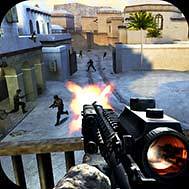The image captures a high-action moment from a first-person shooter video game, featuring a detailed scene of combat within a desert-like courtyard reminiscent of the Middle East, potentially Saudi Arabia. In the foreground, a hand in a camouflage outfit grips a large black automatic machine gun with a prominent scope. The gun is actively firing, evidenced by the vivid burst of flames from its muzzle. The weapon appears to be mounted or steadied on a wooden fence with three visible posts.

In the background, the courtyard is characterized by sand-colored buildings, and notably, one white structure stands out. A palm tree inserted in the upper right corner enhances the desert theme. The courtyard is animated by three to four dark, armed figures, likely soldiers, who are scattering and attempting to escape the gunfire. Adding to the chaotic scene, a visible explosion—represented by red or orange flames—seems to have erupted from an army vehicle, possibly a tank, suggesting an intense battle scenario. The gunfire is directed towards what appears to be the entrance of a fortress, with the soldiers running amidst the disarray.